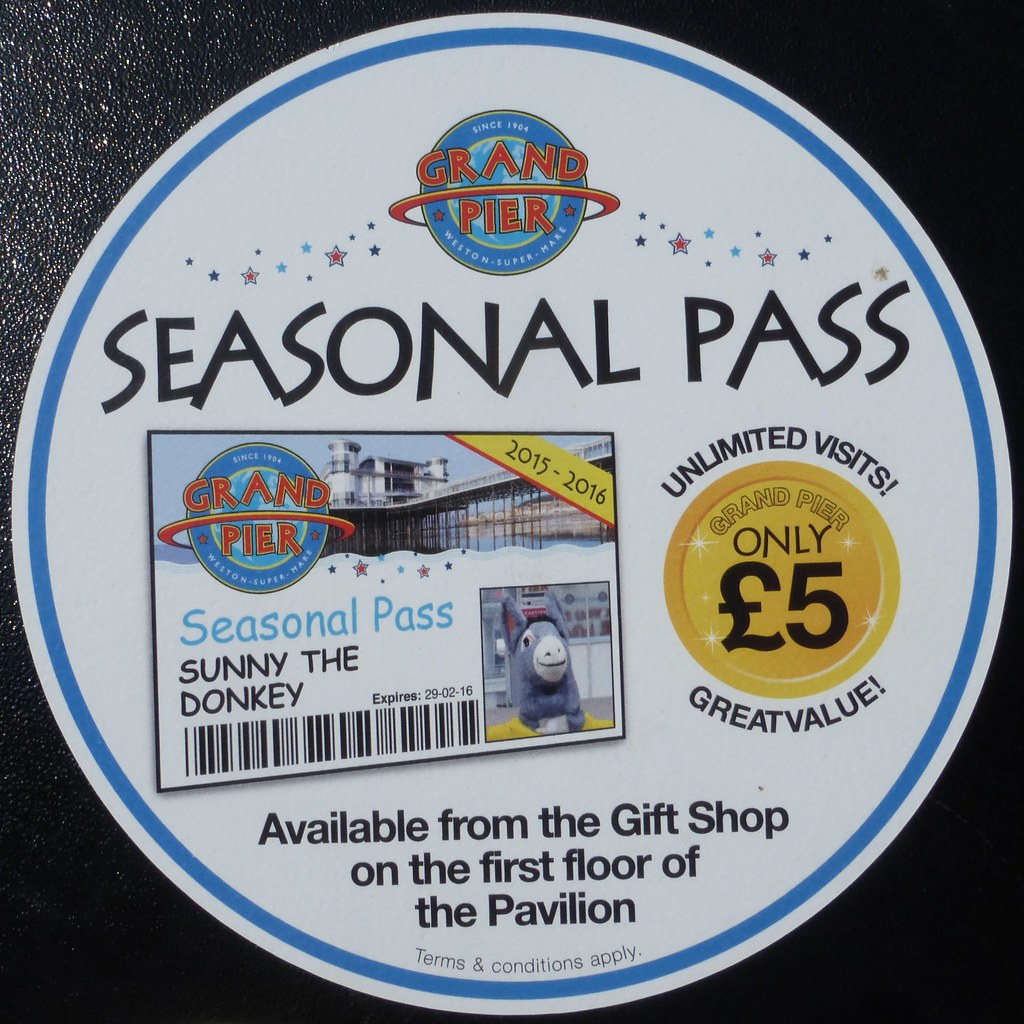The image showcases a promotional sign for the Grand Pier Seasonal Pass. The sign is primarily a white circle framed with blue and encased in black text and graphics. Central to the sign, it reads "Grand Pier since 1904 Western Supermare" with a globe-like logo depicting a blue and green design with an orbiting circle similar to Saturn, and "Grand Pier" in red letters. The emphasis is on the "Seasonal Pass," prominently displayed in black letters along with an illustrative small card of the pass itself. This card includes a picture of Sonny the donkey, the text "Sonny the donkey," and a barcode. The pass also indicates its validity period from 2015 to 2016 and features a yellow background. Additionally, the sign announces that the seasonal pass allows unlimited visits for only £5, making it a great value, and mentions that the passes are available from the gift shop on the first floor of the pavilion. The image integrates all these elements into a cohesive design promoting accessibility and affordability of seasonal visits to the Grand Pier.